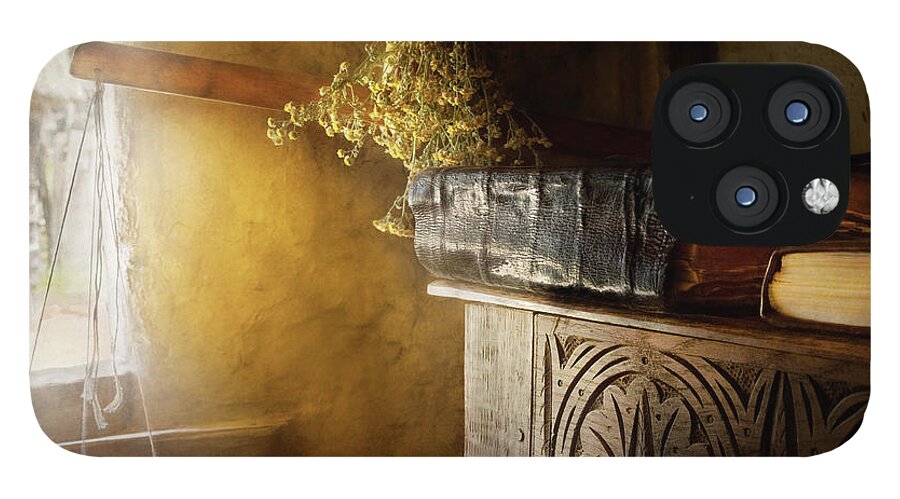The image features a rustic, indoor setting showcasing a large, wooden cabinet or dresser with intricate flower carvings at the bottom. The brown wooden surface of the cabinet holds several items, including two books – a large, thick, black-covered book on the left and a smaller book on the right, positioned with its spine facing left. A tool or device with four circular, lens-like components – possibly camera lenses – is situated above the books.  On the right side of the cabinet, hanging dried flowers can be seen against a crude concrete wall. To the left of the cabinet, there is a window adorned with a dried-looking paper blind that can be lifted or lowered. The window provides a slightly blurred view of a sunny exterior.